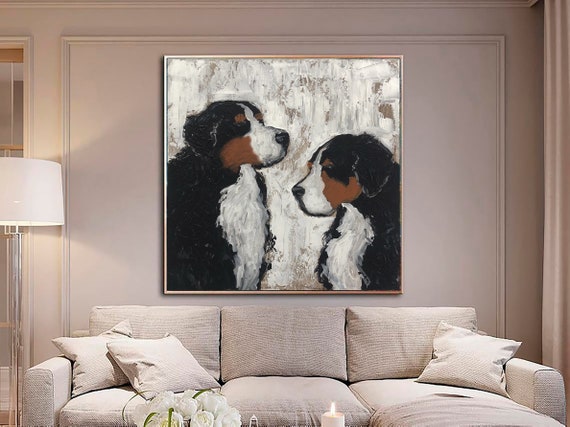In this warmly-lit living room, the walls are painted a bright off-white with a subtle grayish undertone that almost appears white. Centered against the wall is a plush, three-seater couch in a matching off-white color, adorned with three fluffy throw pillows that enhance its cozy appeal. Above the couch, a striking square-framed painting captures attention with its vivid portrayal of two Bernese Mountain Dogs. The dogs, rendered in a raw and expressive style, feature distinct markings: white noses, tummies, and necks, brown streaks on their cheeks and sides of their faces, and black covering their heads and backs. Their lifelike appearance is enhanced by the rough, dynamic brushstrokes that give the painting a vibrant, textured look. The painting's background, also characterized by rough strokes, complements the dogs with a stark white that balances the bold colors of the artwork. To the left of the couch, a simple white lamp adds a touch of elegance and provides soft lighting, contributing to a serene and inviting atmosphere.